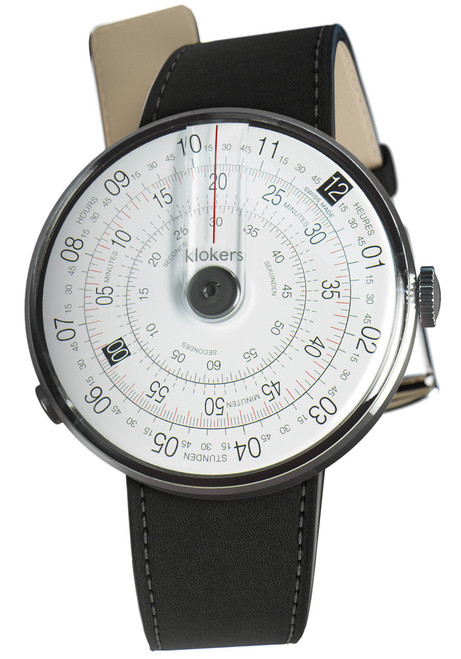In this image, a single, very large wristwatch dominates the frame, nearly filling the entire photo against a solid white background. The watch is meticulously centered, captured in a straightforward perspective that highlights its detailed features. This watch, branded as K-L-O-K-E-R-S, has a striking design with a white circular face. Around the outer rim, standard numerals are displayed, while the inner radial circles feature increments marked from 60 to 05, then 10, 15, 20, and 25, likely indicating an unconventional timekeeping method.

The watch boasts multiple dials and a red hand, adding to its intricate appearance. The watch face includes the text "Swiss Made" below the 12 o'clock position. The outer case of the watch is silver chrome, complemented by a winding mechanism situated on the right side. The band is composed of black leather with contrast beige stitching, and the inside surface of the band is tan. Additionally, the watch features a chrome clasp and a brown loop near the attachment point, enhancing its sophisticated finish.

This image could effectively serve as a promotional piece for a jewelry store, an online retailer specializing in watches, or perhaps a collector's display, showcasing the watch's fine craftsmanship and unique aesthetic.